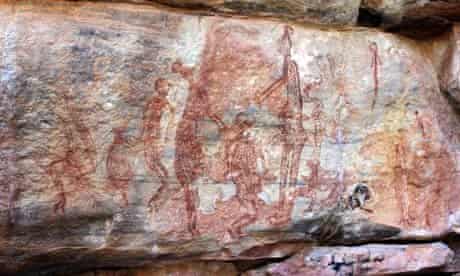The image portrays a large boulder with primitive, Egyptian-style cave paintings on its brown, gray, and orange rock surface. Clearly depicted are six figures, rendered in a reddish pigment that stands out against the limescale-colored wall. The scene shows various individuals in differing positions: some standing, some kneeling. Notably, a central tableau features a kneeling figure in front of a taller figure with outstretched arms, possibly holding an instrument or weapon, while another figure grasps the neck of the kneeling one. Additional figures are arranged in the background, creating a layered effect. The photo, taken from a front view, suggests this may be part of an outdoor setting, possibly within a cave or museum exhibit. Overall, the detailed and vivid depiction conveys a sense of ancient storytelling and ritualistic scene.